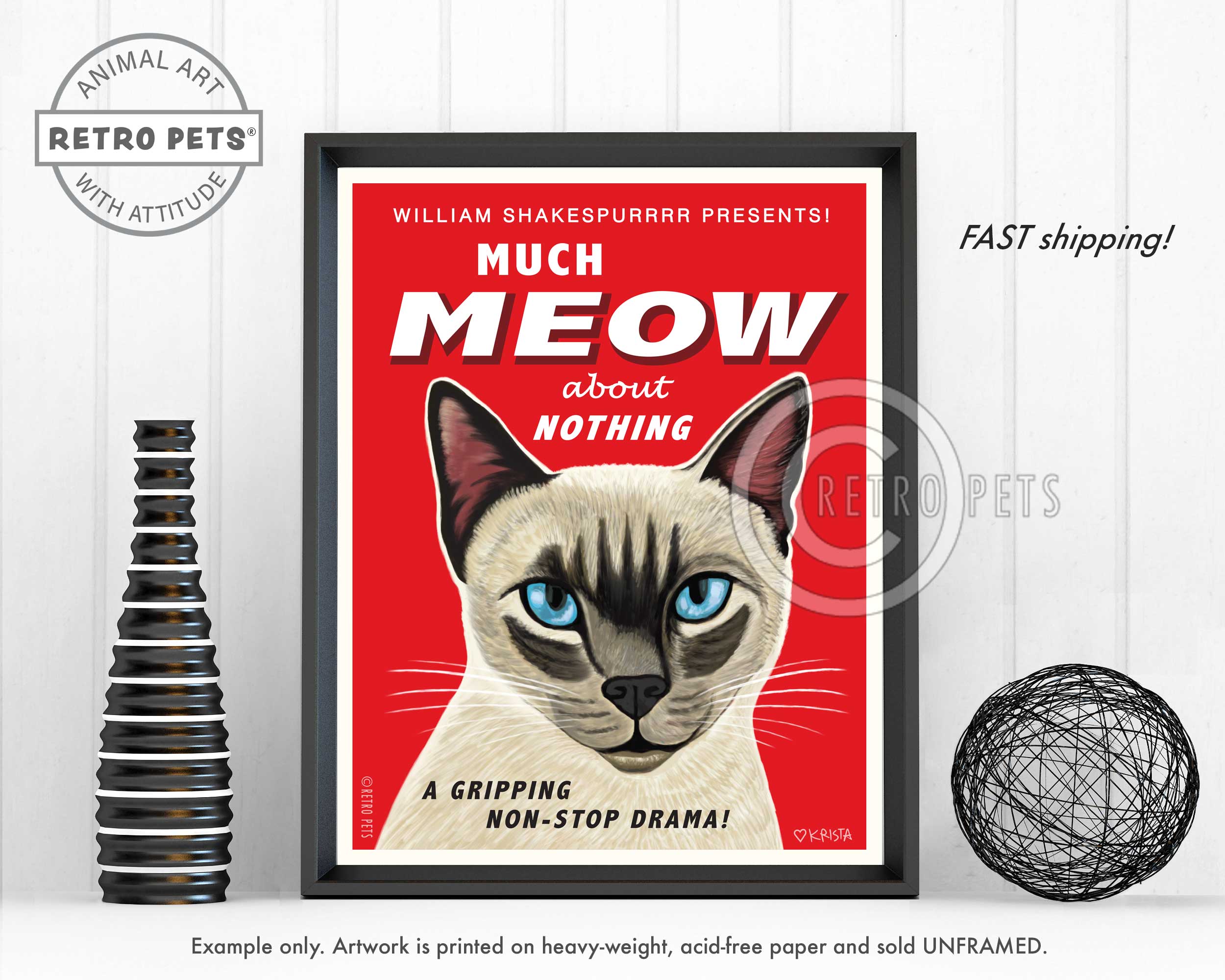The image showcases a detailed scene against a white wood panel wall. In the top left corner, there's an icon featuring the text "Animal Art, Retro Pets with Attitude." Below this icon, there is a black bottle with white rings wrapped around it. On the right side of the image, there's a metallic ball, intricately webbed with thin pieces of wire. Adjacent to this, text reading "Fast Shipping" is prominently displayed.

The centerpiece of the image is a framed artwork with a black border and a white rim, set against a striking red background. The artwork displays the whimsical caption, "William Shakespeare presents Much Meow About Nothing – A Gripping Non-Stop Drama." The portrait is of a Siamese cat with a distinctive appearance: a pale beige coat with darker gray accents under its blue eyes and along its nose, dark gray on its ears, and pink shading inside its ears. In the bottom right corner of the artwork, the name "Krista" is written alongside a heart symbol.